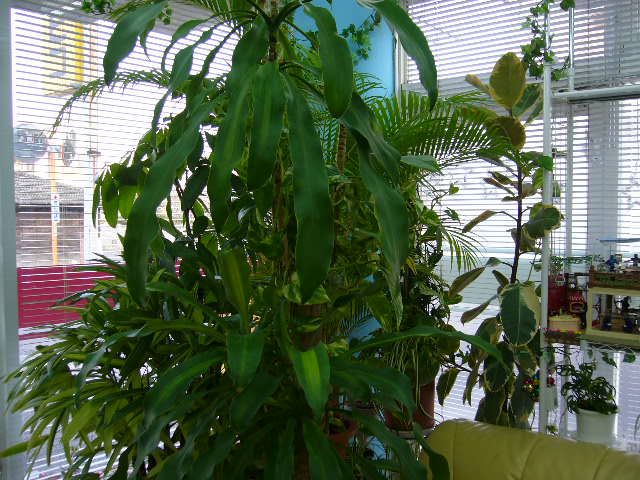This detailed image depicts an indoor room corner showcasing a variety of plants. The scene includes a large plant with lush green leaves prominently positioned slightly to the left, accompanied by several smaller plants. These plants are situated next to a white shelf, which holds various items: a white pot containing a plant on the bottom shelf, a small tray with what appears to be little bags or other small items on the second shelf, and an empty top shelf. Flanking this corner, two large windows are fitted with open blinds, revealing a view outside. Through the left window, a white building with red walls, a darker red fence below, and a small yellow sign with letters, perhaps "C" and "S," are visible. The right window does not provide a clear view outside but rather shows a bit of cab and shelving. The entire corner is painted a light blue, adding a serene backdrop to the indoor greenery. A cushioned chair sits nearby, enhancing the cozy atmosphere of the space.